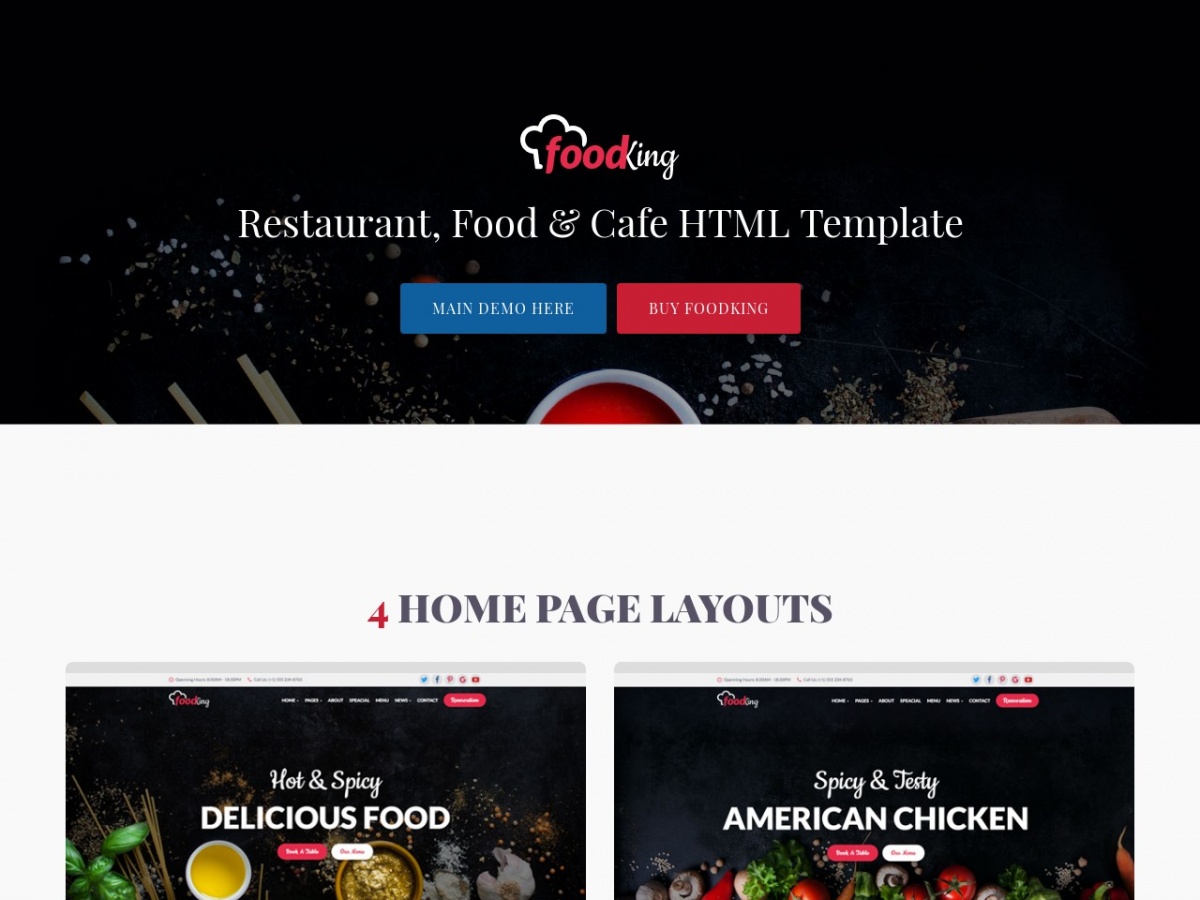The image appears to depict a website design mockup intended for a food-related business named "Food King." The design includes a black navigation bar at the top featuring the logo: "Food King," where "Food" is written in red and "King" in white, with the letter 'D' in "Food" forming the upper stroke of "King." The logo is highlighted by a white chef's hat graphic. To the left of the navigation bar, there's a section labeled "Chopstick Sean," and in the center, a small icon of a bowl of soup.

Beneath the navigation bar, the website is introduced as a "Restaurant, Food, and Cafe HTML Template." Below that, a blue tab labeled "Main Demo" can be clicked for a demonstration, and there's also a red button to "Buy Food King," which although it might sound confusing, likely refers to purchasing the website template.

The main section of the design features a white space highlighting "Four Home Page Layouts," with the word "Four" prominently written in red. This section showcases various design options with headings such as "Hot and Spicy Delicious Food" and "Spicy and Tasty American Chicken," suggesting an emphasis on diverse culinary themes for the Food King brand.